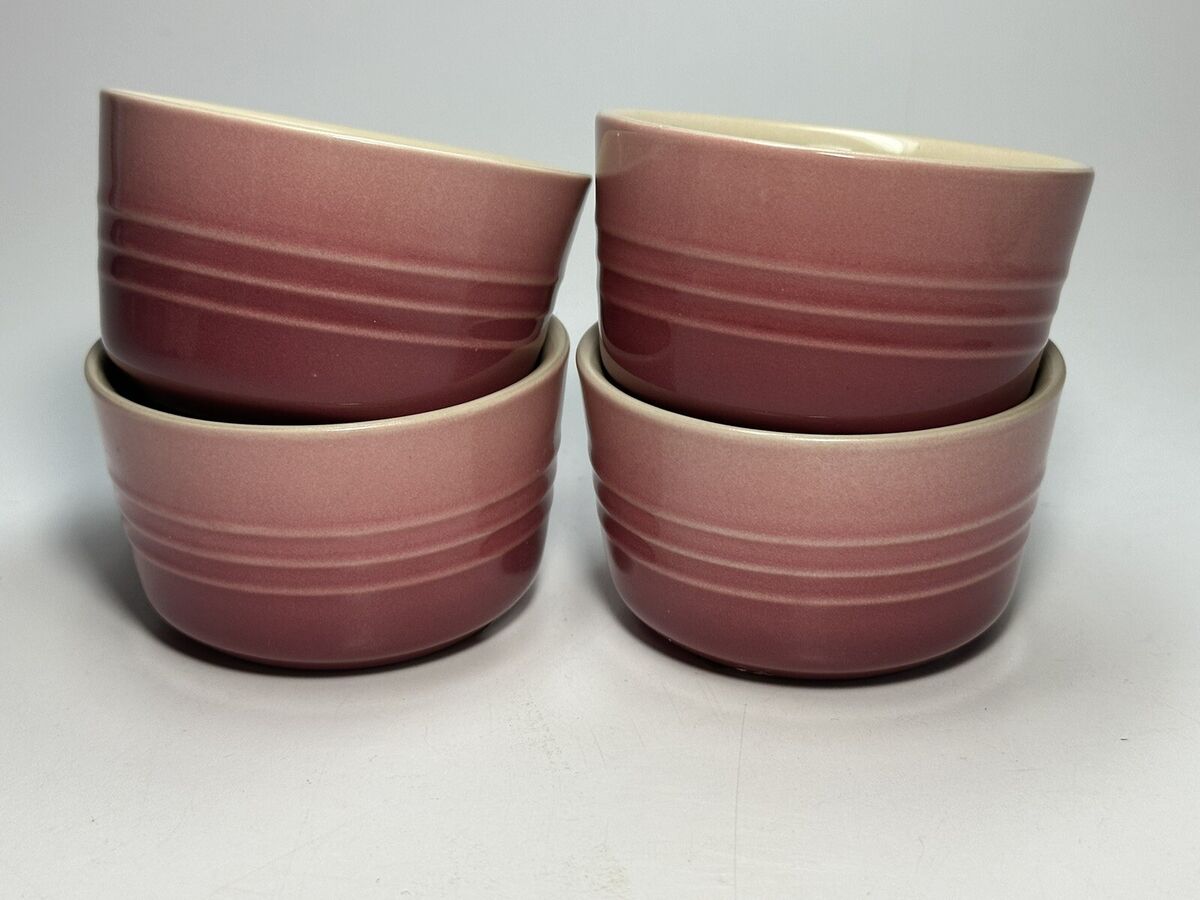The image depicts four short, round ceramic bowls with a ramekin-like appearance, arranged in two neat stacks of two bowls each against an abstract grey background. The bowls, each featuring a creamy-white interior, have an exterior color gradient that transitions from a deep maroon at the bottom to progressively lighter shades of pink as it reaches the top. They are adorned with three light-colored, seemingly raised bands around their middle, providing a visually textured pattern. The bowls atop each stack are tilted slightly to the right, revealing their light cream-colored interiors. Shadows cast by the bowls blend smoothly into the background, creating a cohesive and elegant display.